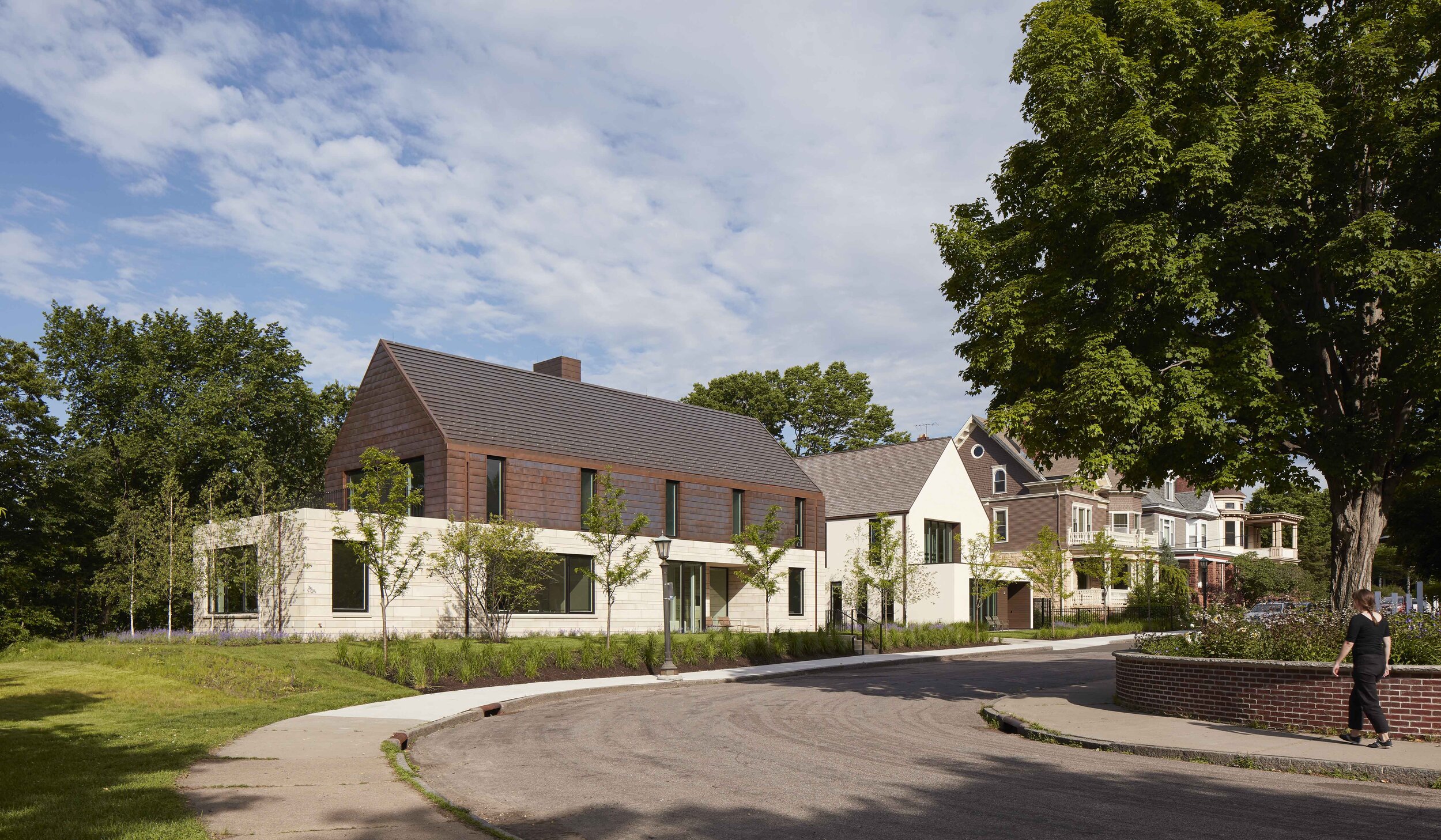The color photograph captures a tranquil daytime scene in a modest yet well-maintained residential neighborhood. The sky is light blue with plenty of white clouds scattered across it. Four houses, characterized by their triangular-shaped dark slate gray rooftops and cream-colored brick borders, line a curved gravel road. The homes, which feature large windows, are set against meticulously groomed light green lawns and are surrounded by both young sapling trees and more mature, towering trees with lush, dark green leaves. 

On the right side of the image, a large tree stands prominently next to a brick retaining wall about two feet tall. A woman dressed entirely in black, of European descent, walks along the sidewalk near this tree. Throughout the neighborhood, additional large green trees offer a verdant backdrop, emphasizing the leafy, serene environment. The residential setting exudes a peaceful ambiance with its harmonious blend of greenery and carefully designed home exteriors.